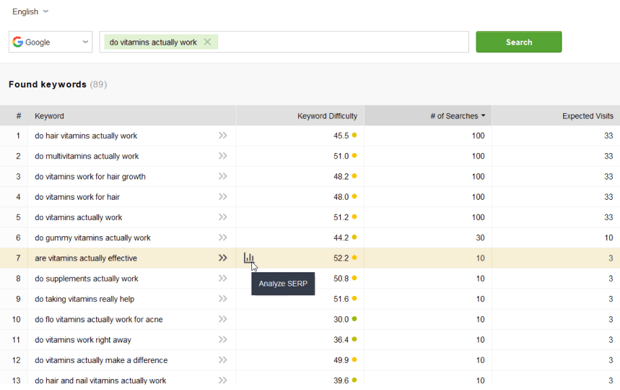The image displays a keyword research tool interface against a white background. In the upper left corner, there is black text resembling a drop-down menu currently set to "English." Below this, another drop-down menu is labeled "Google." Further down, a search bar is highlighted in a yellowish hue containing the query, "do vitamins actually work." To the right of the search bar, a green button inscribed with the word "Search" in white text is present.

To the right side of the interface, there is a gray background section featuring several data points. In black text, it reads "Found keys," followed by the number "89" in gray text. Below this, headings such as "Keyword," "Keyword Difficulty," "Number of Searches," and "Expected Visits" are displayed.

The keyword phrases related to vitamins are listed, including "do hair vitamins work," "do multivitamins work," and "do vitamins work for hair growth," among others. One phrase, "are vitamins actually effective," is highlighted in orange. Additional phrases explore various aspects of vitamin efficacy, such as "do supplements actually work" and "do vitamins work right away."

Keyword difficulty ratings range from 39.6 to 55.2, the number of searches spans from 10 to 100, and expected visits range from 3 to 233. There are no additional elements or text in the image, concluding the information displayed.